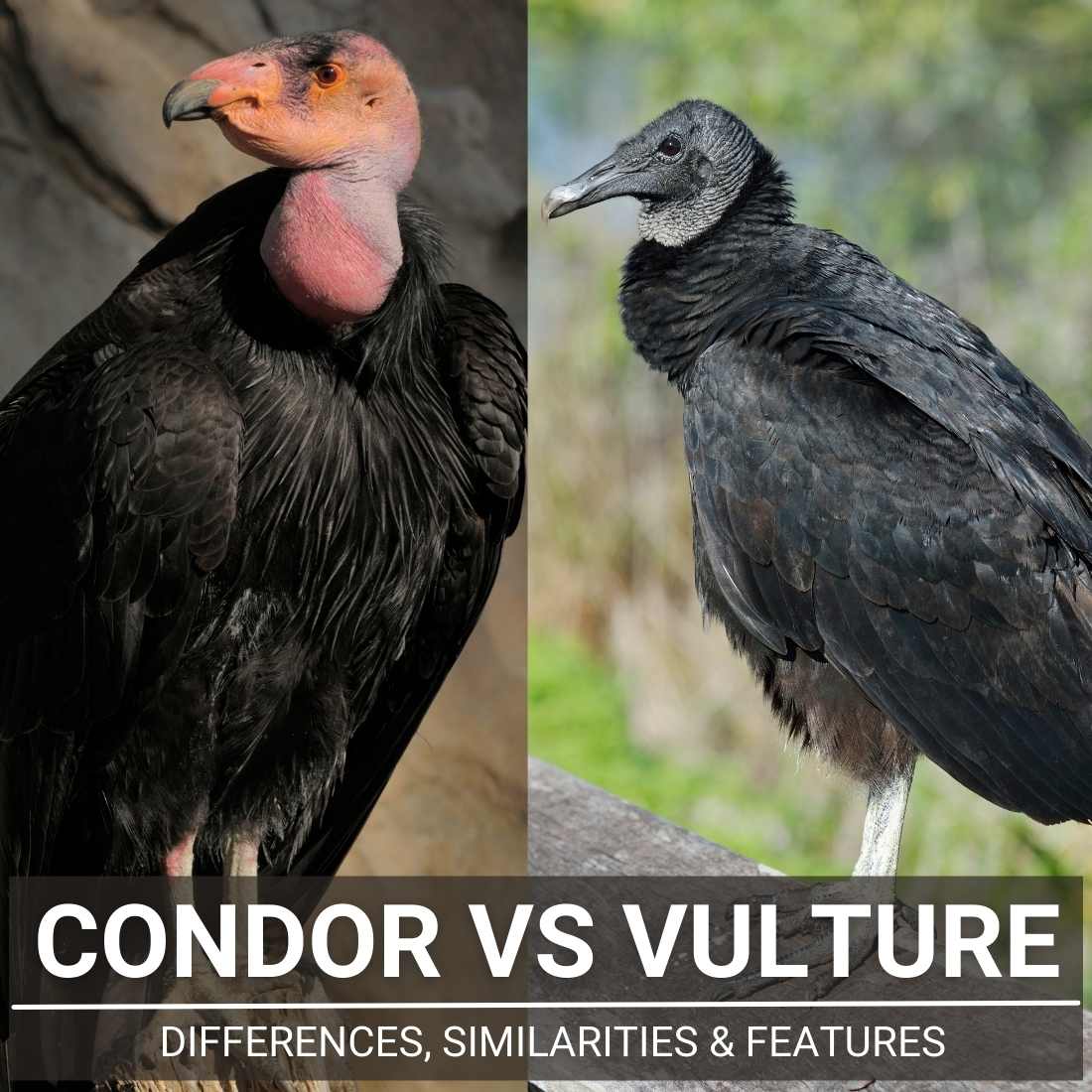The image consists of two side-by-side pictures of birds, showcasing a condor and a vulture, under bright natural outdoor lighting. The left-hand side features a bird with a striking red face and neck, a dark brown eye with a black patch, and predominantly black feathers. Its feet are a dim reddish hue and it stands in front of a tan, rocky formation that provides a shaded contrast. The right-hand side depicts a bird with a black face and neck, black feathers, and white feet, standing on a brown log against a blurred green background, suggesting grass and trees. Both birds are oriented to look towards the left. At the bottom of the image, on a gray background, white text reads "Condor versus Vulture: Differences, Similarities, and Features" with a horizontal white line separating the title from the subtitle.